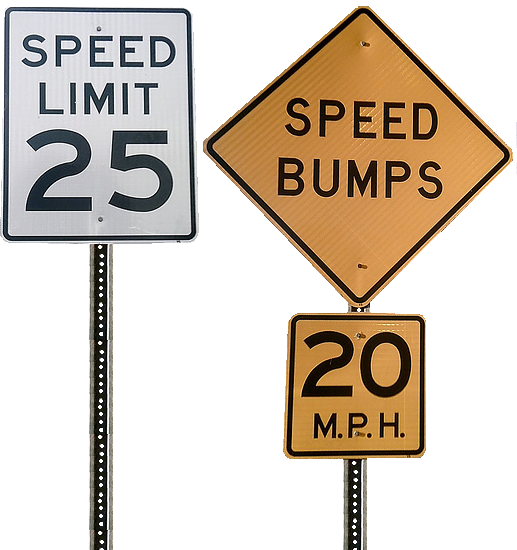The image depicts two distinct road signs set against a solid white background in a square format, characteristic of Photographic Representationalism Realism. On the left, a vertical steel post supports a white rectangular sign oriented in portrait mode, featuring black text that reads "Speed Limit" at the top and "25" in large, bold numbers at the bottom. On the right, a second steel post supports two signs: a yellow diamond-shaped sign at the top with the black text "Speed Bumps," and directly below it, a yellow rectangular sign displaying "20 MPH" in large black letters. Both signs are sharply captured and well-spaced apart, emphasizing the clear, informative nature of these road indicators.